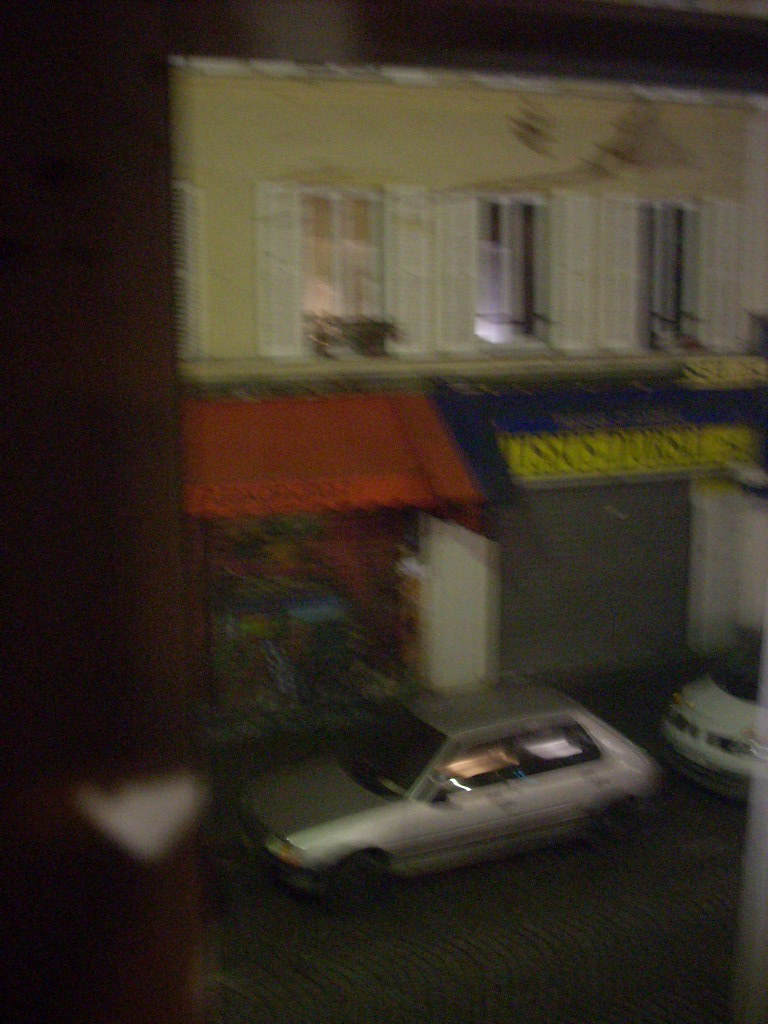The image depicts a vertical rectangle that is noticeably out of focus, creating a blurry and unclear scene. In the background, we see a predominantly brown area at the top, extending down the left-hand side. A distinctive white triangular scratch is visible towards the bottom left. As we move down the image, gray pavement appears, distorted with wavy lines due to the blurriness.

In the mid-ground, an old building reminiscent of a small-town main street captures attention. The upper part of the building features yellow-painted walls with white shutters, accented by some black markings. White trim outlines the architectural details, though the blurriness conveys a shaken appearance.

Below, a red awning suggests the presence of a storefront. A mural appears to be painted on a protective gate beneath the awning. Adjacent to this, there is a blue and yellow sign above a gray garage door that is shut. On the street in front, a couple of cars are parked, contributing to the scene's urban yet nostalgic feel.